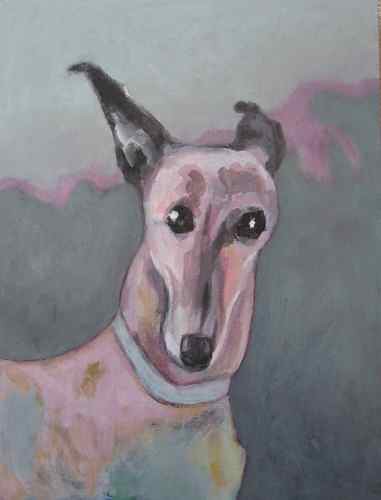The artwork features a stylized image of a dog set against a predominantly gray background, which varies from a lighter shade at the top to a darker shade at the bottom. A pink, squiggly line traverses the upper third of the image, possibly suggesting abstract elements like mountains or other natural forms. The dog, positioned in the lower-left corner, is depicted from the shoulders up, showcasing its pointy black ears—each with white inner patches—one perked up and the other slightly flopped backward.

The dog is characterized by its narrow, elongated face, which is adorned with black eyes featuring white spots, a black nose, and a unique coloration that blends brown and white hues. Its coat at the bottom shows hints of orangish and grayish hair. The dog also sports a light blue collar, adding a contrasting pop of color. In the background, indistinct wavy lines suggest the presence of dark bushes or trees, adding depth to the composition despite its overall low resolution. The artwork merges a blend of abstract and tangible elements, creating an intriguing and detailed portrayal of the dog.